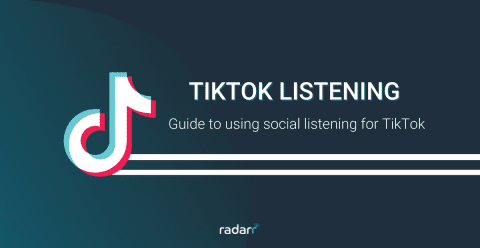A rectangular banner in landscape format displays the TikTok logo prominently. The logo, featuring a musical note with blue and pink outlines, is accompanied by white text. The primary text reads "TikTok Listening," with additional subtext below stating "Guide to Using Social Listening for TikTok." Both lines of text are set against a dark gray background and are underlined by two thin white lines that are half the thickness of the TikTok logo. Centered at the bottom of the rectangle is the word "radarr," written in lowercase white text and spelled uniquely with a double 'r' at the end.